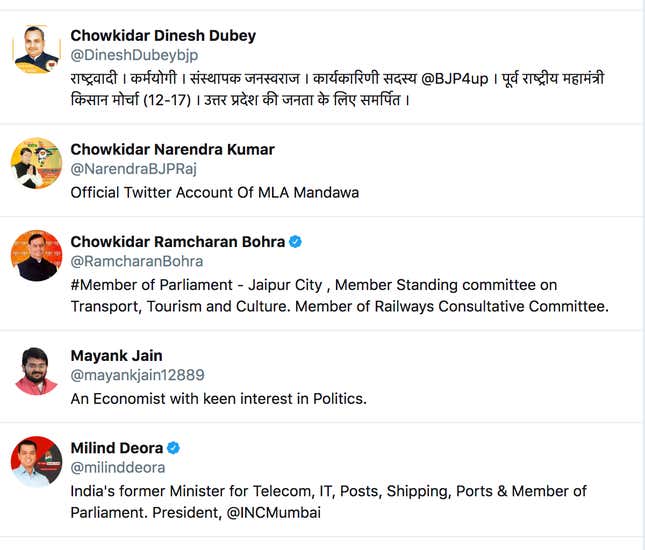This image is a vertically oriented screenshot featuring a list of individuals associated with Indian politics. The source of the screenshot is unclear, as it could be from either a cell phone or a laptop. The image is composed of a grid of white rectangles, which blend into the predominantly white background. Each rectangle is separated horizontally by thin, light gray lines, with a slightly darker, bluish-gray line along the right-hand border of the screen.

The list includes five individuals, each occupying one rectangular box. Each box contains a circular headshot on the left, followed by the person's name in bold black text, their social media handle in light gray, and a brief description of their role or affiliation.

1. **Chowkidar Dinesh Dubey (@DineshDubeyBJP):** Description appears to be in Hindi.
2. **Chowkidar Narendra Kumar:** Official Twitter account of MLA Mandawa.
3. **Chowkidar Ramcharan Bohra (B-O-H-R-A):** Contains additional details, though not specified here.
4. **Mayank Jain (J-A-I-N):** Further description provided in the image.
5. **Malin Deora:** Includes a description of their role or affiliation.

Each entry meticulously follows this format, providing a structured overview of the individuals and their political affiliations.